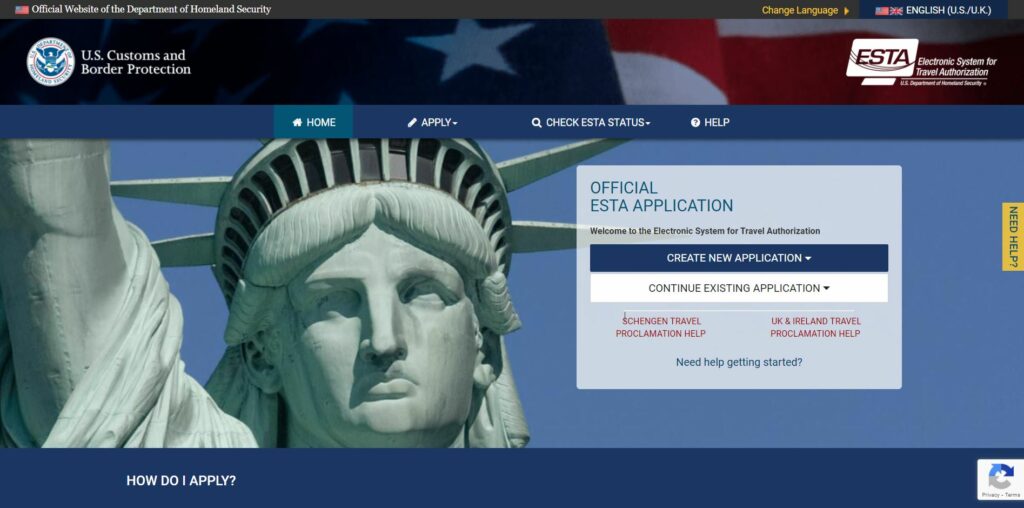A screenshot of a website with a wide aspect ratio, approximately twice as wide as it is tall, depicting the official website of the Department of Homeland Security. The top 5% of the image features a gray navigation bar running horizontally, with a small American flag in the upper left-hand corner. Adjacent to the flag, in white text, is the statement, "Official website of the Department of Homeland Security." On the upper right-hand corner of the gray bar, yellow text reads "Change Language," accompanied by an arrow pointing to the right. Next to this, white text labels an American flag and a British flag with "English (US/UK)" in parentheses.

Below the gray bar, a section with a background of the American flag—stars on the left and stripes on the right—occupies about 25% of the image's height. On the left side of this section is a seal, with the text "U.S. Customs and Border Protection" in white text to its right, displayed in two lines.

Further down, a blue navigation bar, which is about twice as tall as the gray bar above, serves as the menu. The menu items include "Home," "Apply," "Check ESTA Status," and "Help," with "Home" currently selected.

In the bottom portion of the image, a banner shows the face of the Statue of Liberty on the left, set against a backdrop of blue sky. The overall design conveys a formal and authoritative aesthetic consistent with U.S. government websites.